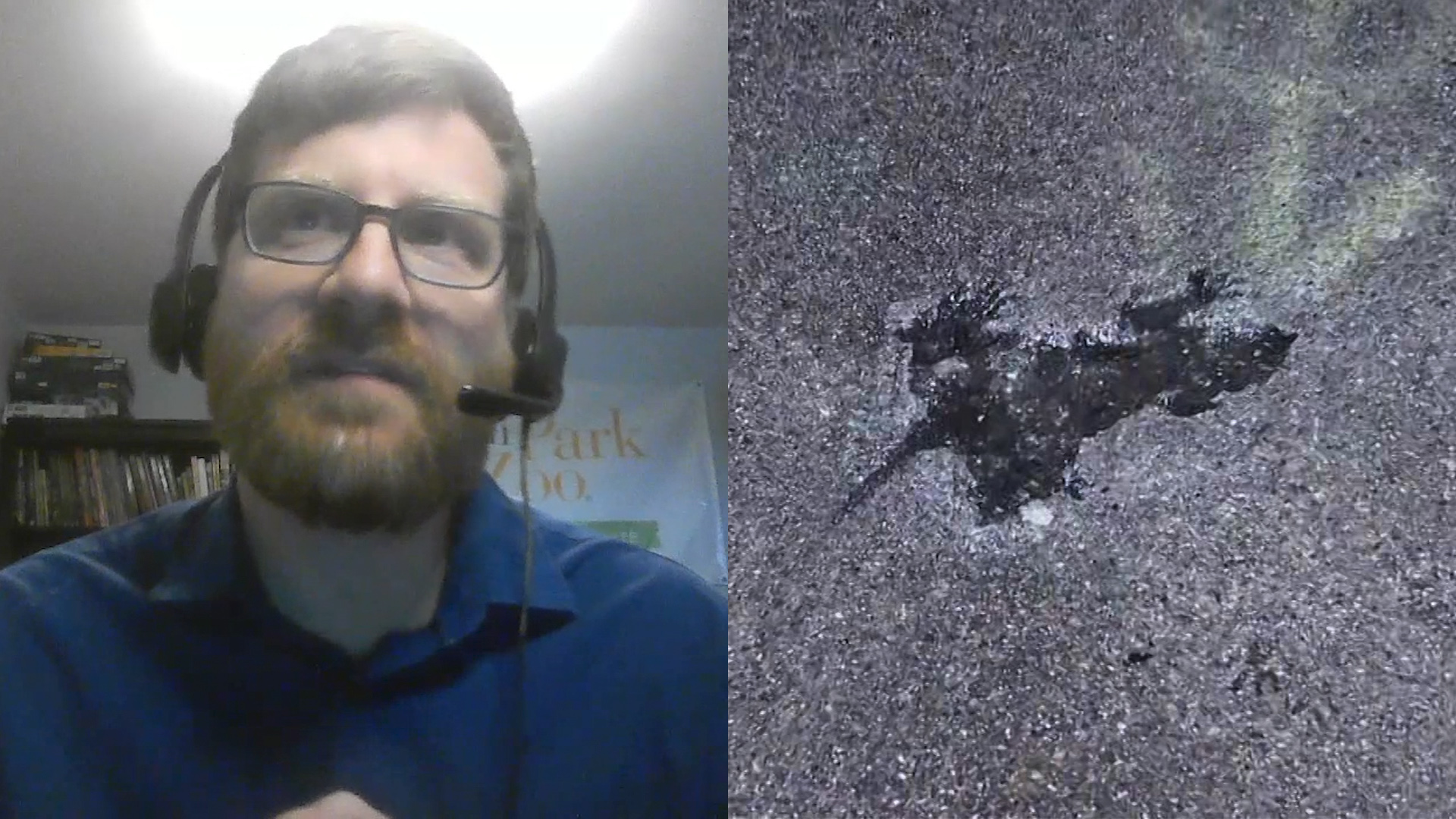The image is divided into two sections. On the left, there's a close-up of a man inside a room. He has brown, slightly reddish hair, a matching beard, and glasses. He is wearing a dark blue button-up shirt and a headset with a microphone positioned near his mouth. Behind him, there's a bookcase filled with books, a poster that appears to include the words "park" and "zoo," and a bright white ceiling light above him. On the right-hand side of the image, there's a murky gray, gravelly or concrete-looking floor with a grainy appearance. In the center, there is an indistinct shape which looks like the imprint of a small animal, possibly a lizard, rat, or mouse. The animal's imprint appears either crushed into the concrete or as if it set while the concrete was still wet.